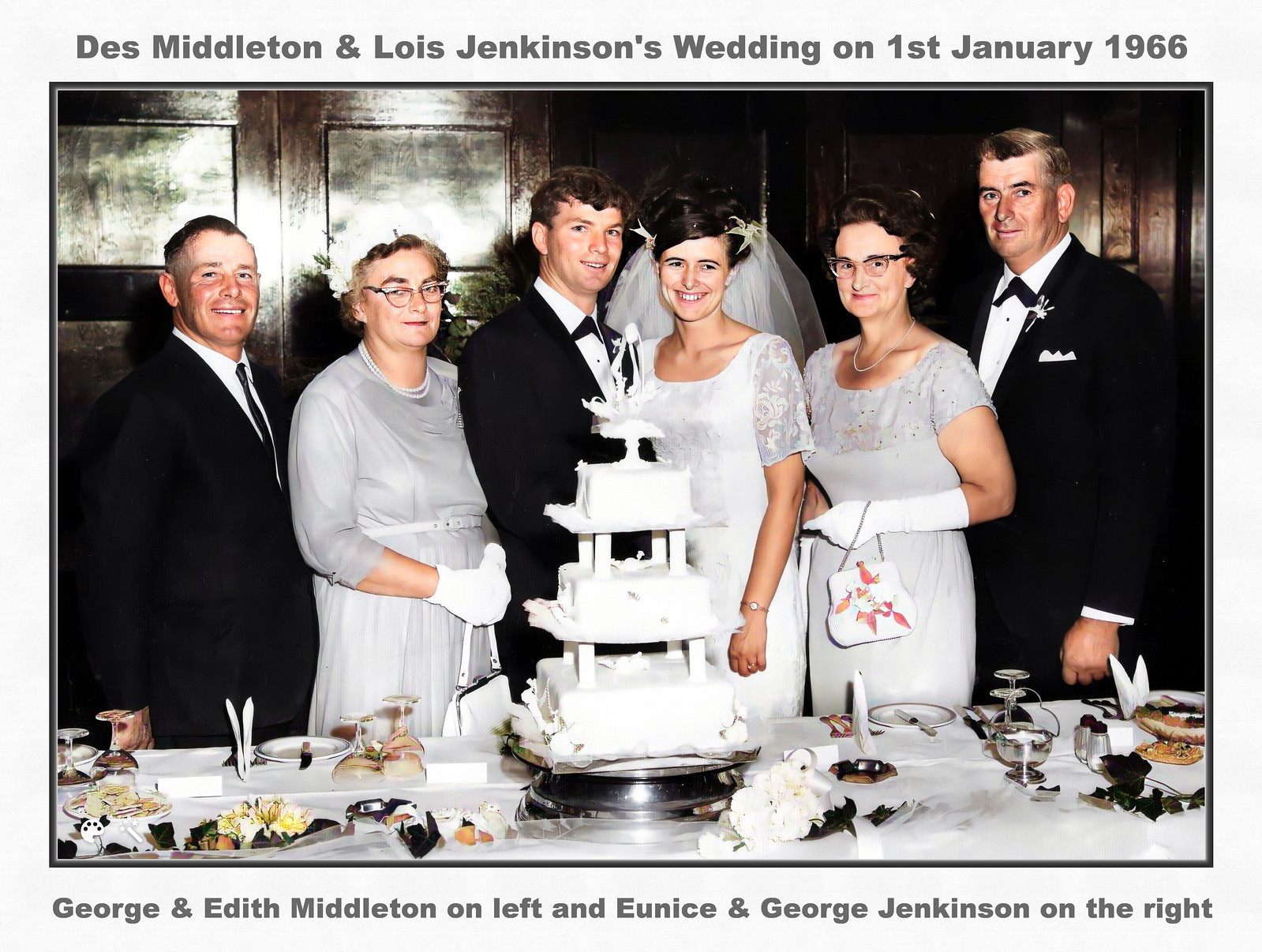This vintage wedding photo, dated January 1, 1966, captures the joyous union of Des Middleton and Lois Jenkinson. Standing behind a grand four-tier wedding cake, the bride and groom are flanked by their smiling parents. The scene unfolds in what appears to be a church hall, characterized by dark wood paneling in the background. 

The bride, adorned in a classic bridal dress with a veiled headpiece, and the groom, dressed in a black suit with a continental tie, take center stage. To their sides stand their parents, formally dressed in period attire. The bride's mother, wearing an ice-blue dress with elbow-length gloves and holding a small purse, stands next to Edith and George Middleton, who are identified at the bottom of the photo. The groom's mother also wears a matching ice-blue outfit, complete with wrist-length gloves and a flowery hat. Both fathers don black suits, with the groom's father wearing a standard necktie.

The table in front of them is elegantly set with a white tablecloth, plates, overturned stem glasses, and an array of flowers, perfect for a wedding banquet. The caption beneath the photograph names George and Edith Middleton on the left and Eunice and George Jenkinson on the right.